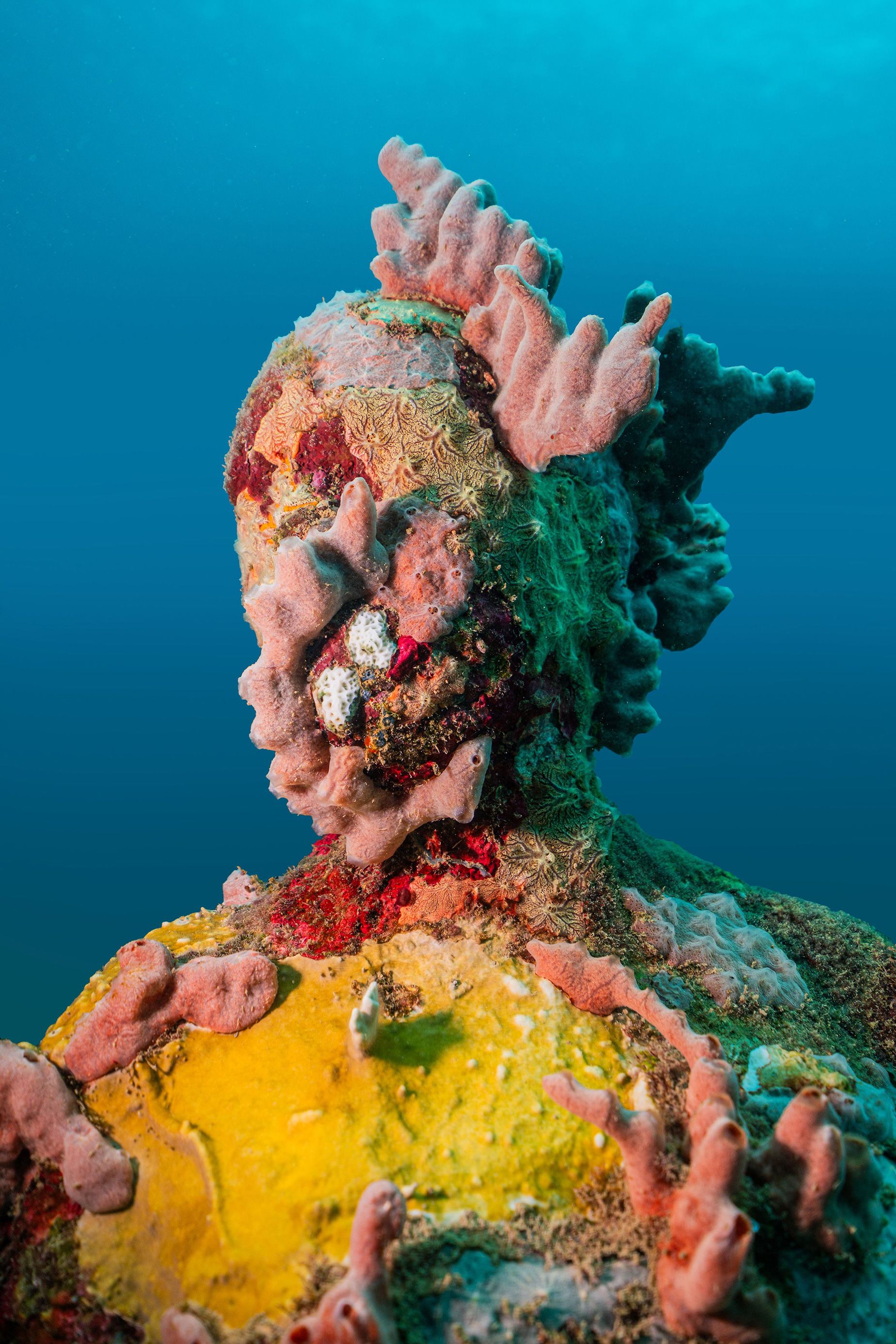This is a photograph of an incredibly intricate piece of coral in the ocean, encapsulated in a vibrant teal-ish blue backdrop. The coral formation strikingly resembles the silhouette of a human, with an oval-shaped head and shoulders, although it is not an actual statue. This remarkable structure is a lush tapestry of colors and textures, featuring a mix of pink, red, yellow, cream, and blue hues. The main focal point is a large, intricate coral that hosts various other coral organisms, creating a rich and highly textured surface. Bright mustard yellow, traditional coral pink, green, bright red, and specks of white can all be seen. Notably, a significant blotch of pink coral adorns what might be perceived as the chest area, with more pink coral growing upwards, enveloping areas where the cheeks or face might be, extending to the top and back of the head. Additional coral pieces jut out from the right side of the structure, adding to its complex and captivating appearance.